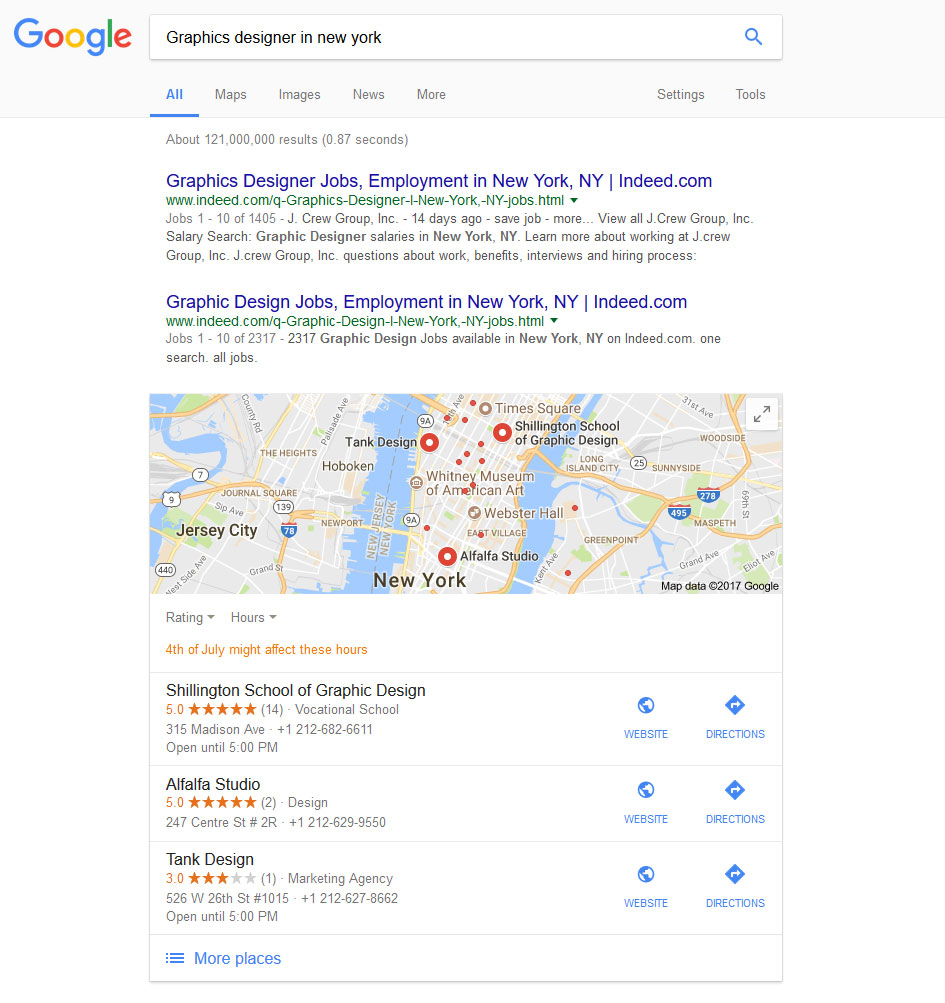The image is a screen capture of Google search results. In the top left corner, the iconic Google logo is displayed in its vibrant rainbow colors. Below the logo, there is a search bar containing the text "Graphics Designer in New York." Just underneath the search bar, there are various category tabs labeled All, Maps, Images, News, and More, followed by options for Settings and Tools.

The search has produced approximately 121 million results in an impressive 0.87 seconds. The initial search results display job listings, such as "Graphic Designer Jobs, Employment in New York, New York" prominently featured on Indeed.com.

A map is also displayed, focusing on the Jersey City and New York area, showcasing several educational institutions related to graphic design. Notable locations include:

- **Shillington School of Graphic Design**: Located at 315 Madison Avenue, this vocational school has received 14 stars.
- **Alpha Studio**: Situated at 247 Center Street, number 2R, this studio boasts a 5-star rating based on 2 reviews.
- **Tank Design**: Found at 526 West 26th Street, number 1015, this location has a lower rating of 3 stars.

Each of these entities contributes to the graphic design landscape in New York, offering both employment opportunities and educational resources.